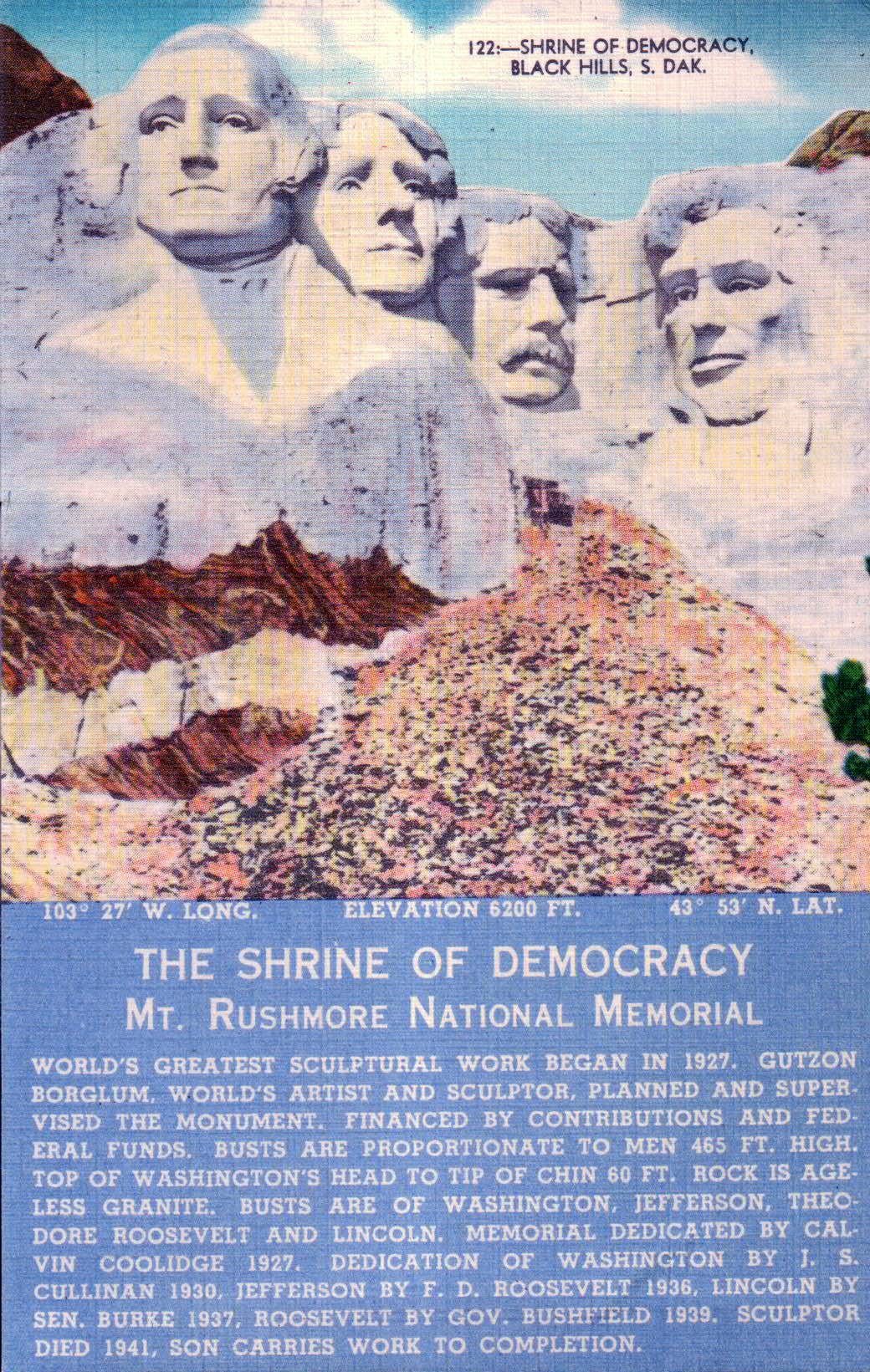The image features a detailed poster of Mount Rushmore with the iconic granite faces of Presidents George Washington, Thomas Jefferson, Theodore Roosevelt, and Abraham Lincoln. Against a backdrop of white clouds and blue sky, the top right corner of the poster displays the title "122-SHRINE OF DEMOCRACY" in bold black lettering. Beneath this, the location is specified: "Black Hills, S.D., Black Hills, South Dakota." 

The poster highlights the rugged terrain below the sculpted faces, showcasing the rubble from the carving process. The lower half of the poster uses a light blue background and white lettering to provide crucial details, such as the geographical coordinates "103 degrees, 27 minutes West Longitude" and "43 degrees, 53 minutes North Latitude," along with the elevation at 6,200 feet.

The poster is titled "Shrine of Democracy, Mount Rushmore National Memorial" and includes an informative description: The monument, often hailed as the world's greatest sculptural work, was initiated in 1927 by artist and sculptor Gutzon Borglum. The project, which stands as a testament to American history and democracy, was financed through contributions and federal funds. It mentions that the busts of the presidents, each proportionate to a height of 465 feet, with Washington's face measuring 60 feet from the top of his head to the tip of his chin, were carved with precision in the easily workable granite.